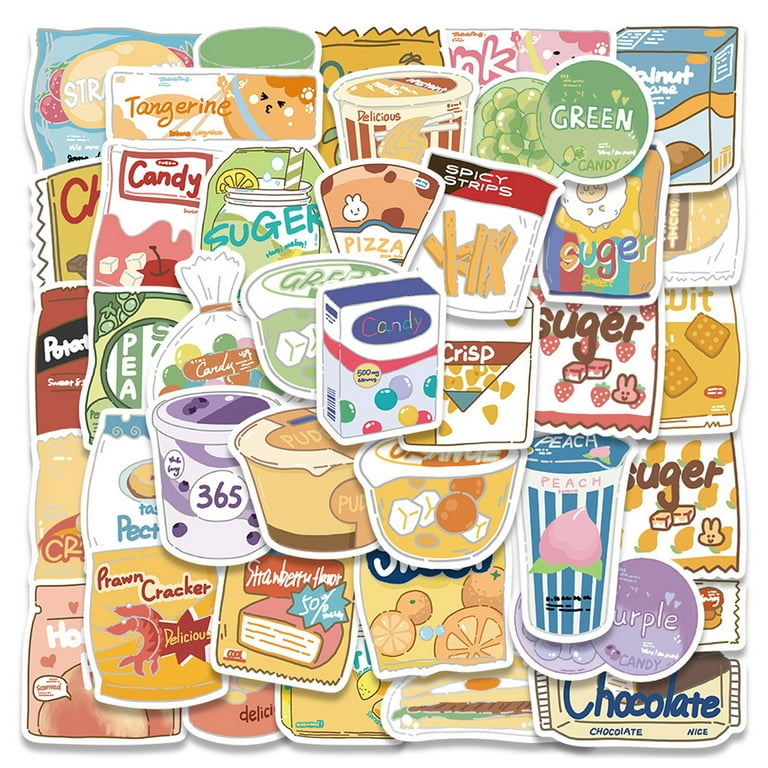The image is a large, animated collage forming a rough square shape, filled with approximately 50 to 100 overlapping cartoon representations of various food items, predominantly sugary treats and snacks. The array of items includes chocolates, prawn crackers, puddings, crepes, candies, spicy strips, pizza strips, tangerine snacks, strawberry-flavored treats, walnuts, green candies, and peach drinks. Each treat comes in diverse packaging forms such as cups, packs, cans, and sachets with vibrant and dimmed colors including red, shades of blue, yellow, orange, purple, brown, and green, reflecting the candy theme.

Centrally located is a box labeled "candy," showcasing multicolored circles. Surrounding it are various shapes: to the upper right, a vertical rectangle labeled "spicy strips" featuring images resembling strips of chicken; adjacent to it, a triangle with a curved top labeled "pizza," displaying a bunny face; in the upper right corner, a circle labeled "green candy." In the lower parts, the left side features a rectangular bag saying "prawn cracker delicious," and next to it, another item labeled "strawberry." The lower right corner has a horizontal bar labeled "chocolate." The objects are arranged in a cluttered yet visually engaging manner, each partially obscured by another, blending into a colorful and whimsical mosaic of treats.